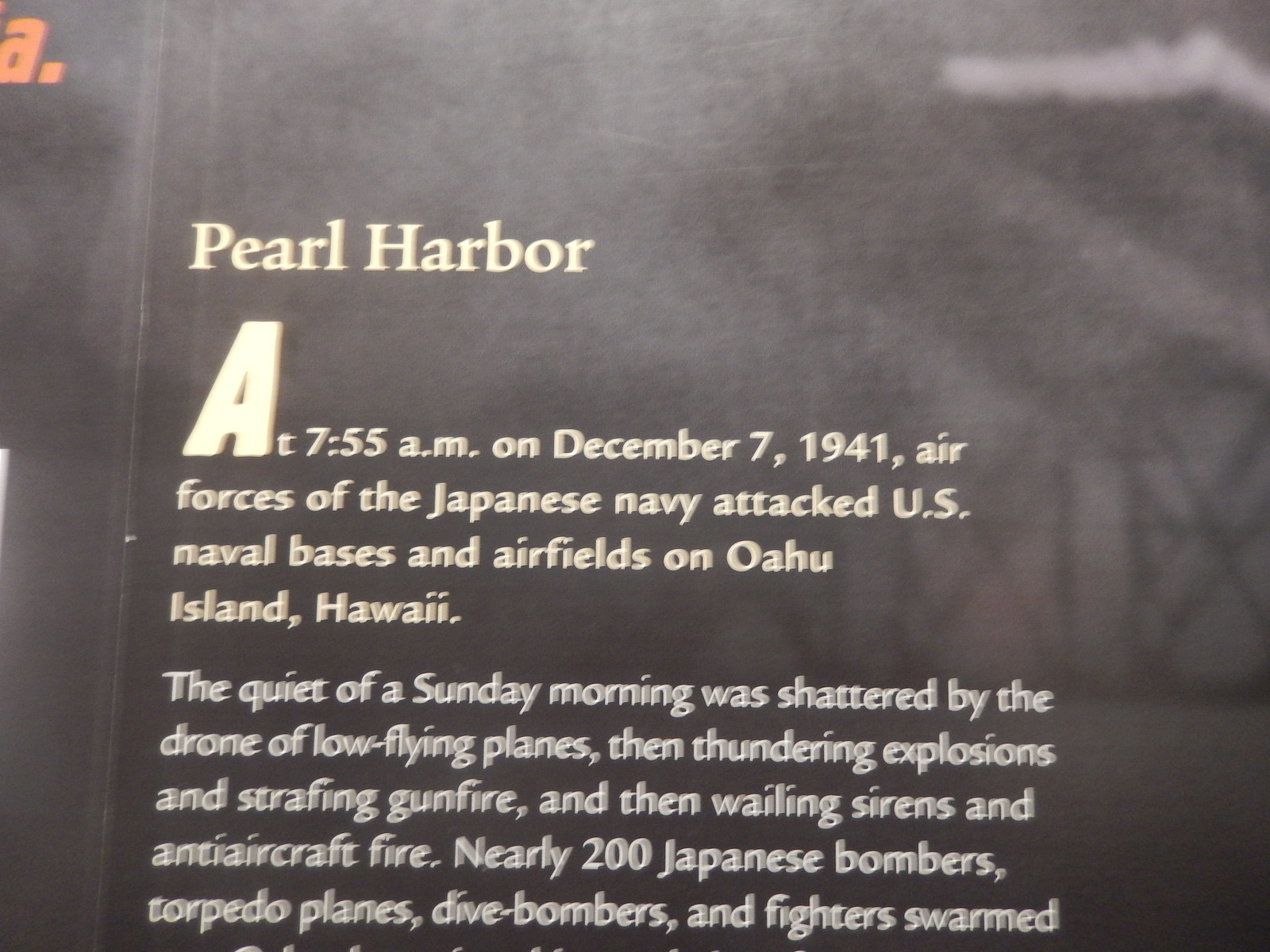The image depicts an informational placard with a solid black background, photographed at a slight angle, causing the words to appear extended towards the top, and captured in a somewhat blurry state. The white font text begins with the title "Pearl Harbor." It narrates the events of December 7, 1941, starting at 7:55 a.m., when Air Forces of the Japanese Navy launched an attack on U.S. naval bases and airfields on Oahu Island, Hawaii. The placard describes how the tranquil Sunday morning was abruptly disrupted by the ominous drone of low-flying planes, followed by a series of thunderous explosions, strafing gunfire, wailing sirens, and anti-aircraft fire. Although the text promisingly mentions nearly 200 Japanese bombers, torpedo planes, dive bombers, and fighters, the lower section of the placard is cut off, leaving the description incomplete. In the upper right-hand corner of the placard, there's a small segment showing some burning ships. The dimensions of the plaque appear to be approximately four inches tall and six inches wide.